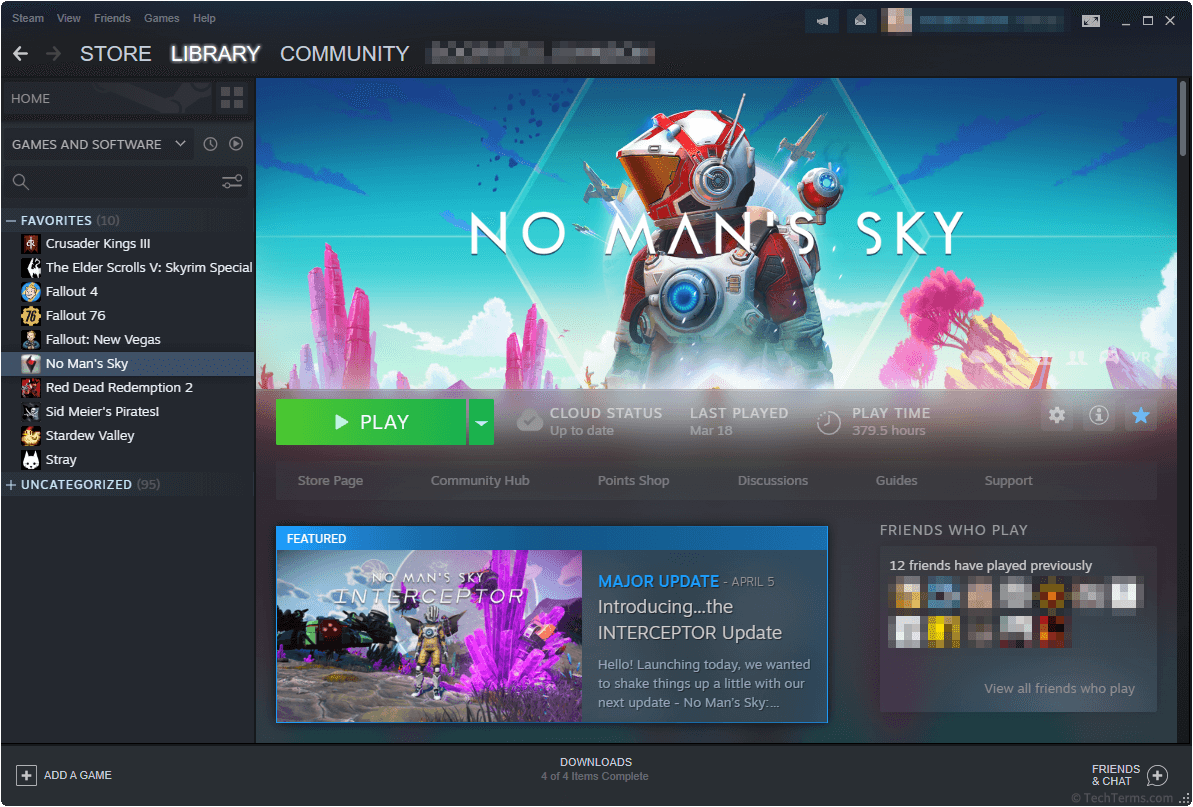A detailed screenshot showcases the main interface of the Steam application, set against a sleek black background. In the upper left corner, a menu bar features small gray text options: Steam, View, Friends, Games, and Help. Just below, more prominent white text highlights the options Store, Library (currently selected), and Community. Dominating the lower right of the screen, a vibrant digital artwork depicts an astronaut dressed in a white helmet and a white and red spacesuit. The background is a dazzling, futuristic landscape with pink, cavern-like mountains, flower trees, and a turquoise sky. In the bottom-left corner of this artwork, a green play button is positioned next to gray text detailing the game’s status: "Cloud Status: Up to Date," "Last Played: March 18," and "Playtime: 379.5 hours." To the far left of the screen, a navigation bar is visible, guiding users through different application sections.